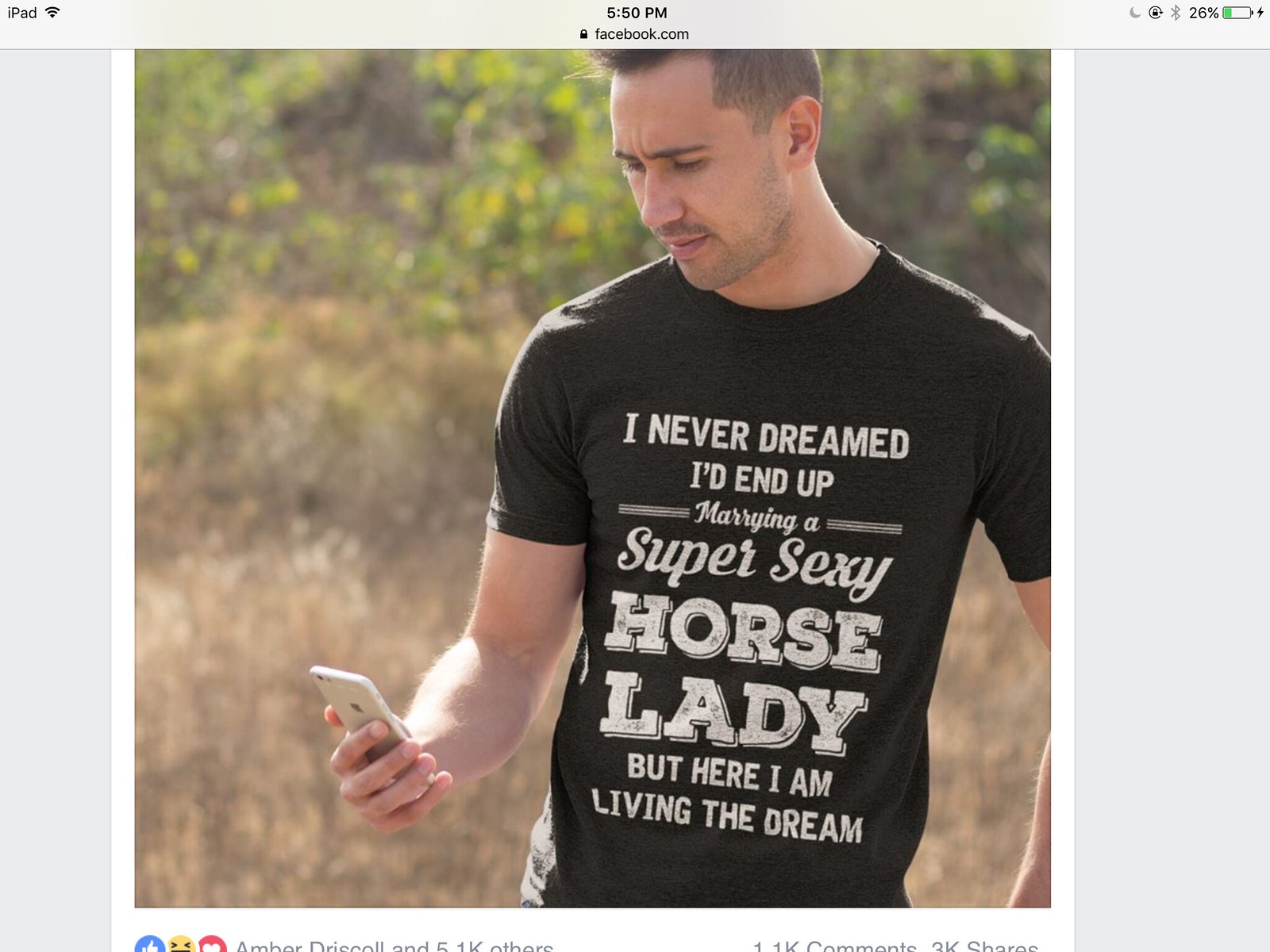The image is a screenshot from an iPad, displaying the Facebook.com website at 5:50 p.m., with the battery at 28%. The post captures a photo of a relatively attractive, clean-cut man with dark brown hair and a slight mustache, looking down at his iPhone. He is outdoors, with a background of out-of-focus green trees. The man is wearing a black short-sleeved T-shirt with white lettering that reads, "I never dreamed I'd end up marrying a super sexy horse lady, but here I am living the dream." The photo is cropped from the waist up, preventing a view of his pants. There's some cut-off writing below the image.